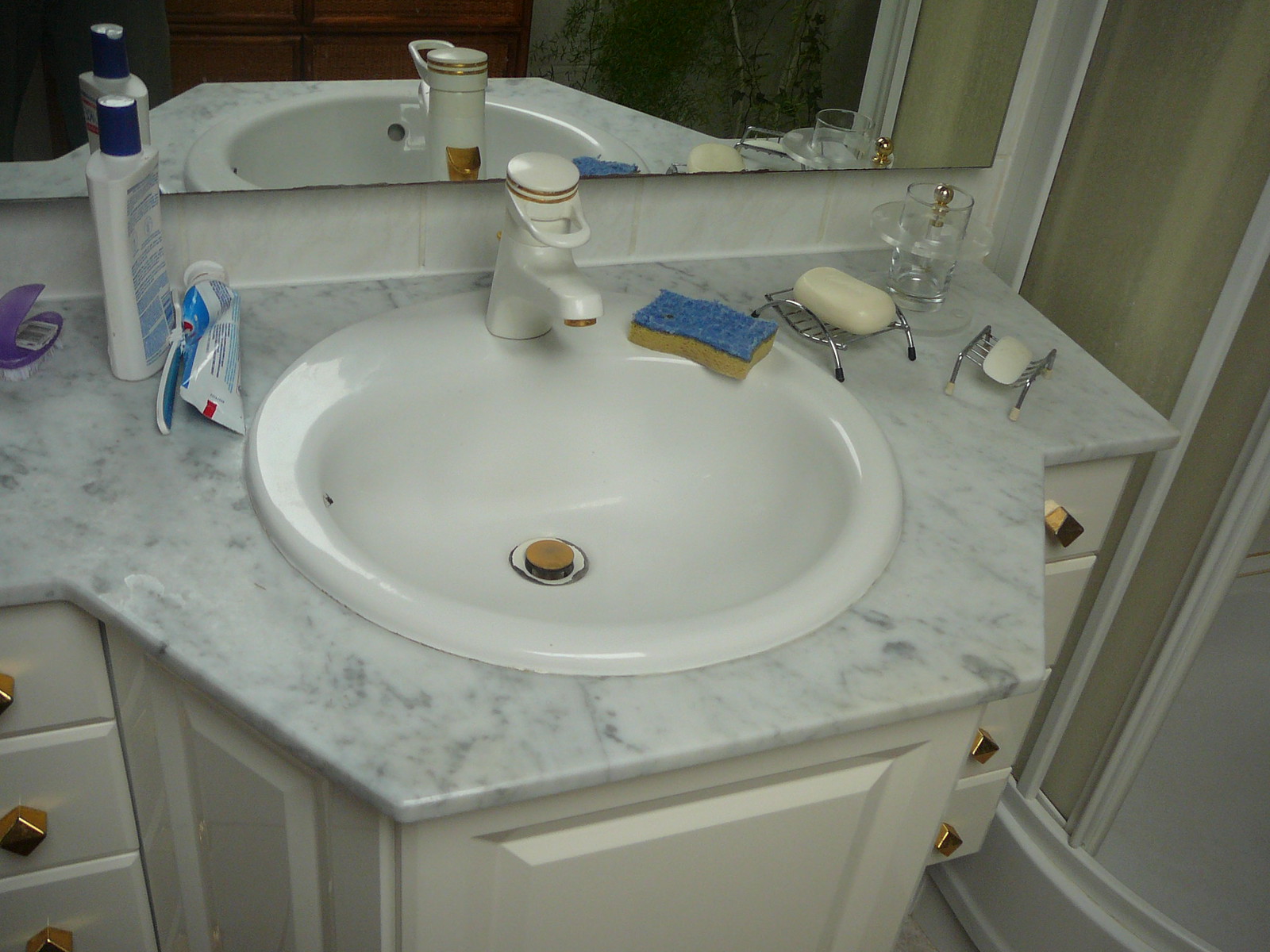The image captures a section of a meticulously organized bathroom. Dominating the scene is a large mirror that spans the length of the back wall, reflecting a gleaming white faucet with intricate gold trim. On the counter, which is adorned with an elegant mix of white and gray marble, sits a variety of toiletries. There are two tubes of toothpaste, one in blue and white, and the other predominantly white with a hint of red. A bottle of lotion with a blue top, a small purple container, and a dual-colored sponge, blue on one side and yellow on the other, add a splash of color. An assortment of soap is neatly arranged in metal holders—one holding a larger white bar, the other a smaller piece. A glass, perched in a silver stand with a gold-accented top, sits next to these items.

Beneath the counter, a pristine white cabinet is flanked by drawers on both sides; three on the left with gold handles, and four on the right. The open shower doors reveal a clean bathtub, completing the picture of this well-maintained bathroom.